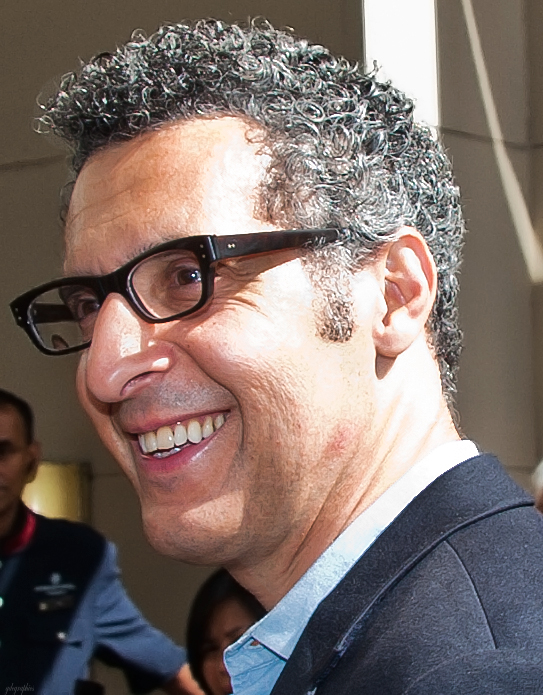The image is a close-up of John Turturro, who is dressed in a black suit jacket with a blue undershirt and small, thick-framed black glasses. His short but curly hair, once dark, is now turning gray. John is looking to the left of the image with an open-mouthed smile, and sunlight illuminates the left side of his face, suggesting the photo was taken outdoors. In the background, partially obscured by John, is a person in a black jacket adorned with an insignia, their arm raised. Additionally, there is a blurry, dark-haired woman who appears either distressed or frowning, but her expression is difficult to discern due to her position and the image's focus on John.